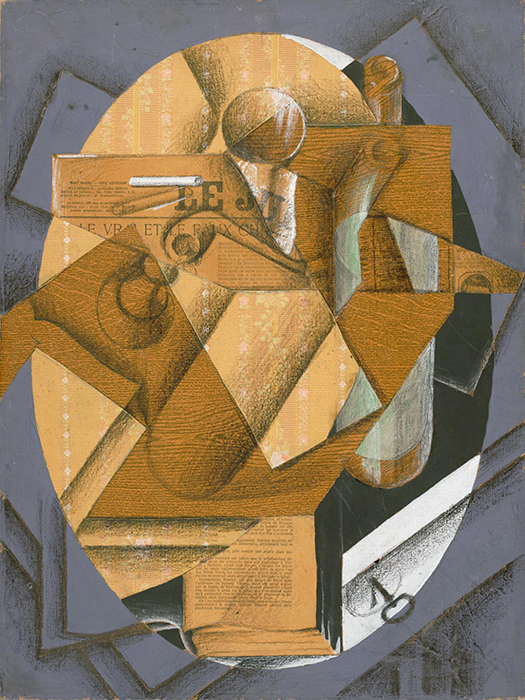This captivating piece of abstract art is a masterfully layered collage, set against a dark gray background and showcasing an intriguing amalgamation of geometric shapes and intricate textures. Dominated by an oval-shaped centerpiece, the composition features a variety of beige, black, white, and earthy brown tones. Towards the lower right corner, flat, gray wooden boards are stacked, tinged with hints of brown. Above this, at the six o'clock position, sits an open antique book adorned with visible text and surrounded by the oval frame, transitioning from white to black and then beige. Adding to the complexity, the artwork incorporates elements of a skeleton key, blending seamlessly with the layered patterns. The artwork also includes depictions of newspapers, magnifying glasses, and various motifs like smoking pipes and bowls, all rendered in shades of gray, white, and a spectrum of browns—from pale to medium and burnt sienna. With its meticulous blend of textures and hues, the piece evokes a sense of depth and layered storytelling, making it an enthralling modern art composition.